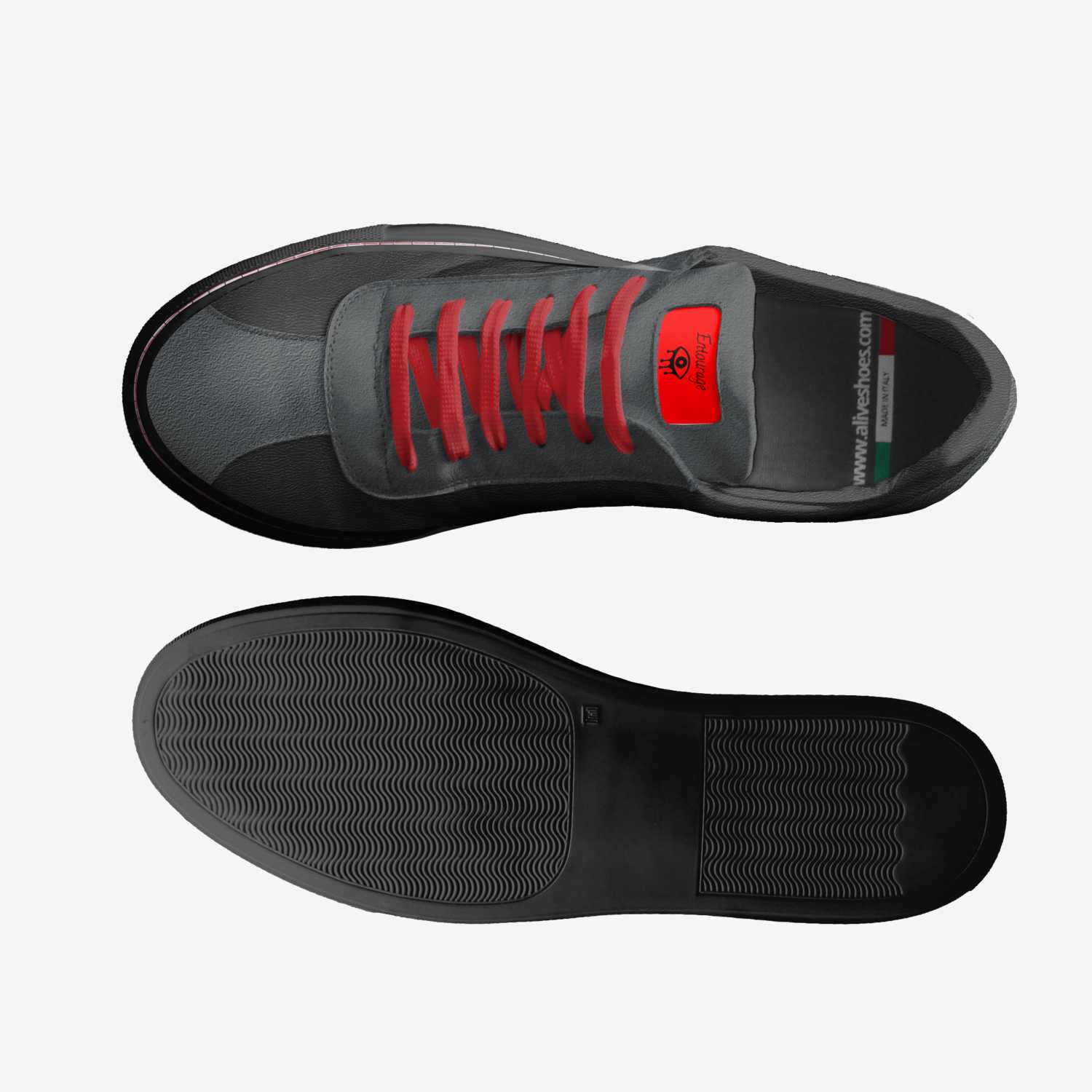On a light gray background, the image features a pair of gray shoes with distinctive red shoelaces. The top shoe, which is the right foot, is positioned upright and facing to the left, revealing a gray tongue and a red label on the tongue with a black eyeball design, dripping black paint, and some text above it. The interior of the shoe displays a green, white, and red stripe resembling the Italian flag and the text "AliveShoes.com" in white. The bottom sole of the shoe is visible, showing a black, wavy grip pattern that provides slight traction, more prominent at the heel and front. Below the top shoe, the left foot shoe is shown upside down, with its black sole visible, emphasizing its smooth central part and wavy tread design at the heel and front.